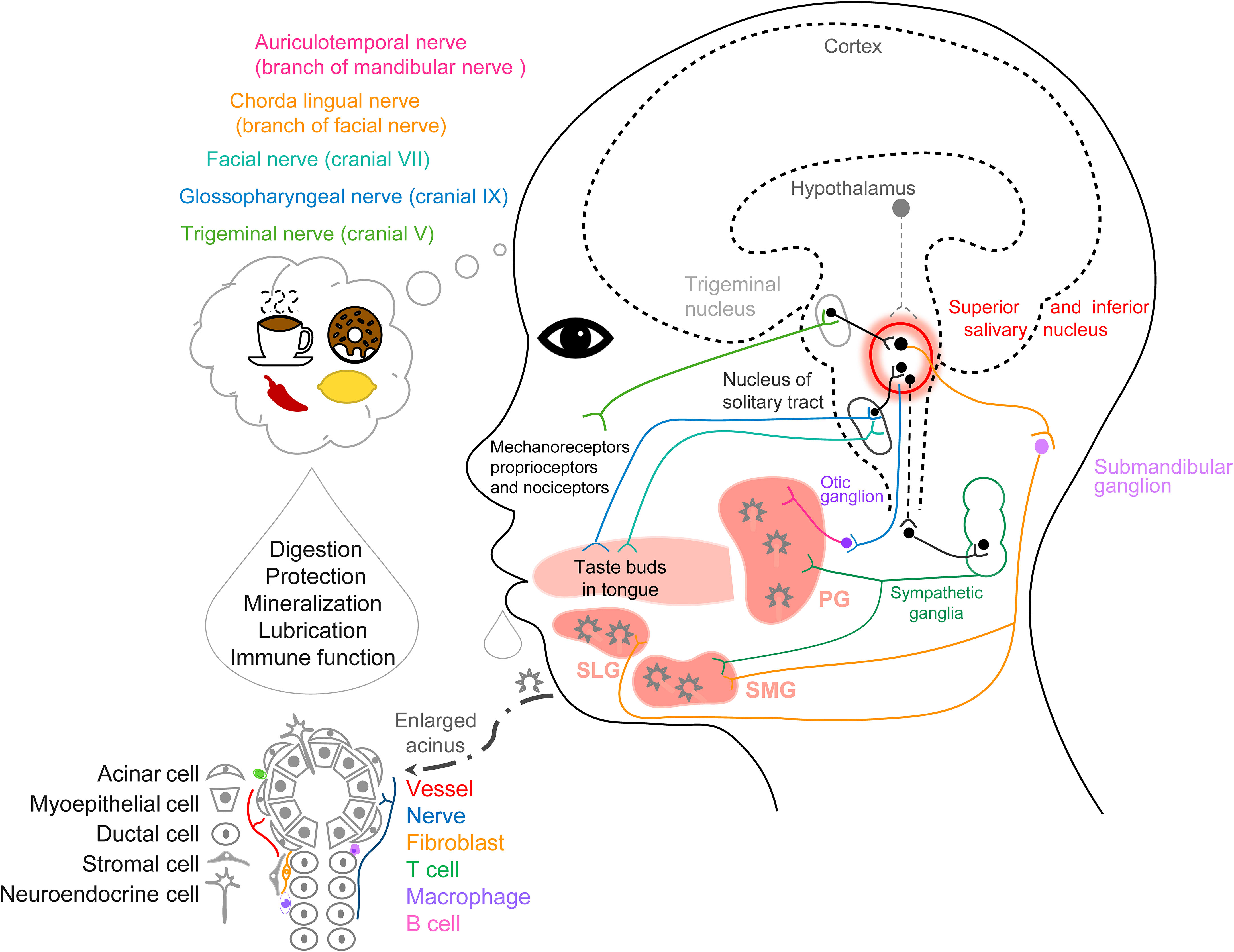This detailed scientific diagram depicts a side profile of a human head and emphasizes the interconnectedness between taste perception and brain function. The illustration shows the brain's cortex, hypothalamus, taste buds on the tongue, various nuclei such as the superior and inferior salivary nuclei, and numerous nerves, including the auriculotemporal, cortolingual, and trigeminal nerves. Colored lines traverse from the taste buds to different brain regions, highlighting neural pathways.

On the left side, a thought bubble contains images of a cup of coffee, a donut, a red chili pepper, and a lemon, indicating the individual's thoughts about these foods. Below this, a textual annotation describes the functions involved in this process: digestion, protection, mineralization, lubrication, and immune function. Additional detailed annotation beneath outlines various cell types, such as myoepithelial cells, ductal cells, stromal cells, neuroendocrine cells, and others, further explaining their roles. This intricate diagram, blending vivid illustrations with comprehensive labeling, appears to be intended for educational use in biology or medical studies, illustrating the complex interactions between taste, neural pathways, and bodily functions.